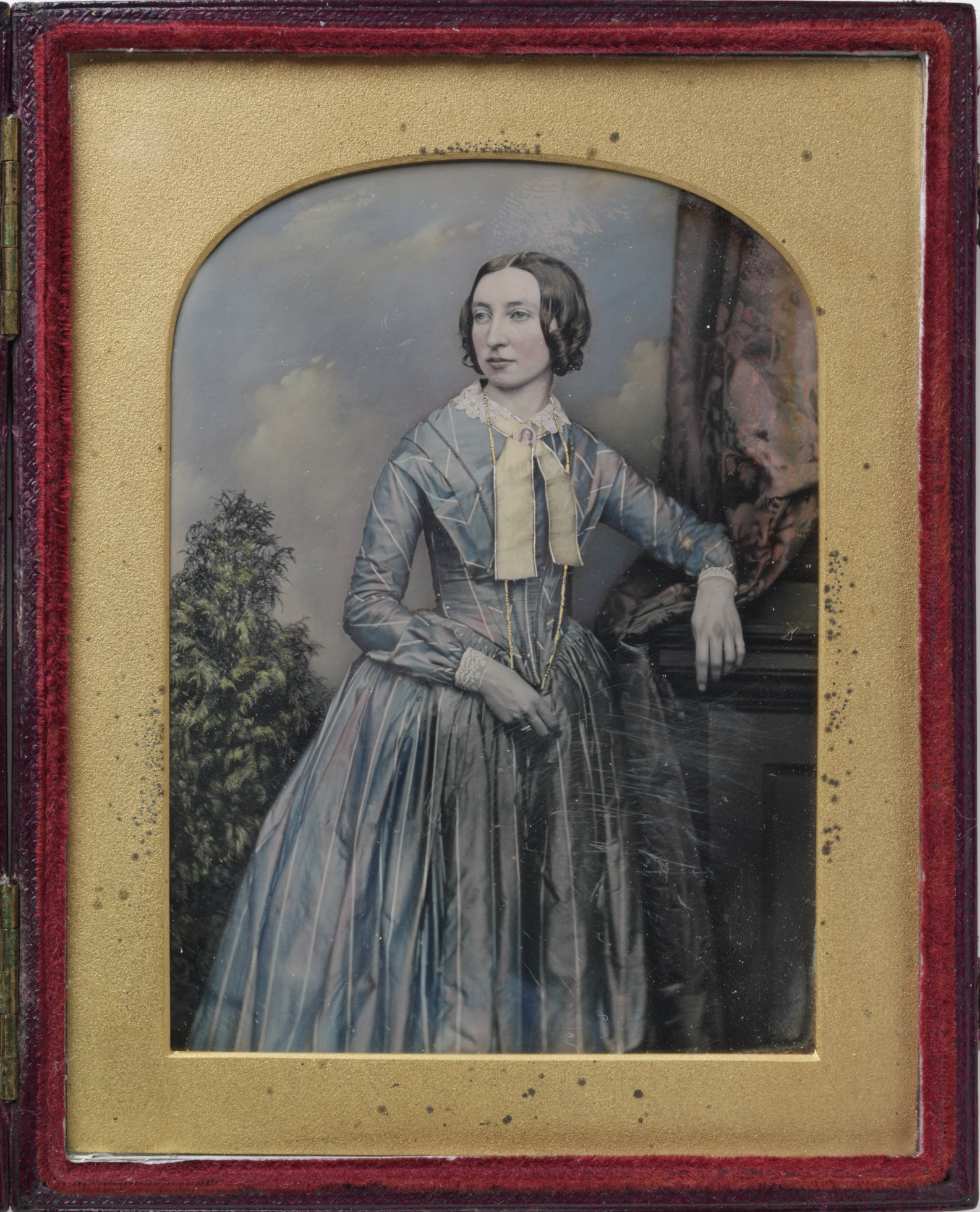This image depicts a painting of a Victorian-era woman in a portrait orientation, set within an ornate frame. The frame is designed to resemble a doorway with a rounded top arch. The mounting board around the painting is gold in color, which is bordered by a red felt section. Encircling the red felt is a thin brown leather outline, completing the edge of the frame. Notably, on the left side of the frame, there are two brass hinges, suggesting that this portrait is possibly part of a cover or a stand, perhaps akin to the top of a box or a picture book.

The female subject of the painting wears a high-collared blue dress embellished with white and pink highlights and white frilly cuffs. The dress features a hoop style from the hips downward, giving it a voluminous appearance, upon which her right arm rests. She has a white trim around her neck and two thick white ribbons hanging from the neckline. A ring adorns her right wedding finger. Her dark hair is styled in tight curls and is tied back, complementing the rosy cheeks that give her a slightly stern expression as she gazes off into the distance to the left.

The background includes a painted blue sky with clouds and a green shrub on the left side, partially cut off. Additionally, her left arm (on the right side from the viewer's perspective) is leaning on dark brown or black furniture draped with a cloth. The painting has a faded quality, adding to its aged appearance.